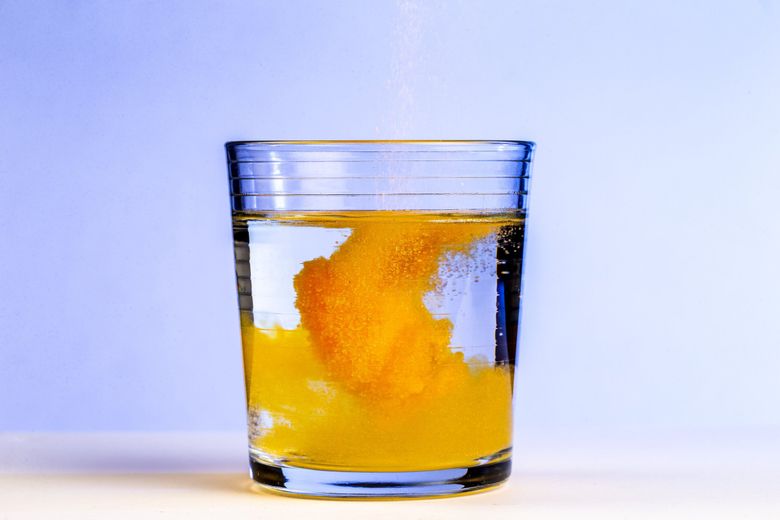This photograph features a clear drinking glass, approximately four to five inches tall, filled to about 80% with water. The glass, which could resemble a wine glass, is meticulously centered on a white tabletop against a light, sky-blue background. The water appears blue due to the background color. Intriguingly, a substantial amount of orange powder has just been added to the water, creating a vivid visual effect. At the center of the glass, a cluster of the orange powder forms a dark, concentrated patch, which gradually disperses into lighter shades of orange towards the sides. This creates a swirling, cloud-like pattern in the water, with the orange color being more intense at the top and thinner at the bottom. Additionally, the glass has four distinctive notches near the top, forming clear rectangular shapes before the rim. The overall composition of the image, devoid of any other text or elements, captures the dynamic interaction between the water and the newly introduced orange powder.